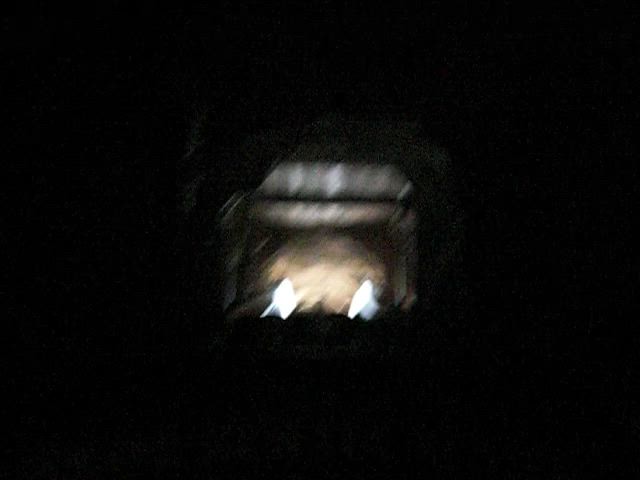This image is quite indistinct and heavily blurred, making it challenging to clearly discern its elements. Dominated by darkness, the focus is on a central object that appears to have a square-like shape with two small lights at the bottom. These lights look somewhat like flames or vehicle lights, but their exact nature is unclear. Behind this central object is a contrasting area with a whitish-brown hue, possibly resembling a rock or another indistinct object. Above these features, there is a ceiling-like structure that appears reflective and metallic, giving the impression of a confined space such as a hallway or the interior of a vehicle. A black pipe or bar runs across this reflective upper area, adding to the sense of an enclosed or mechanical environment.